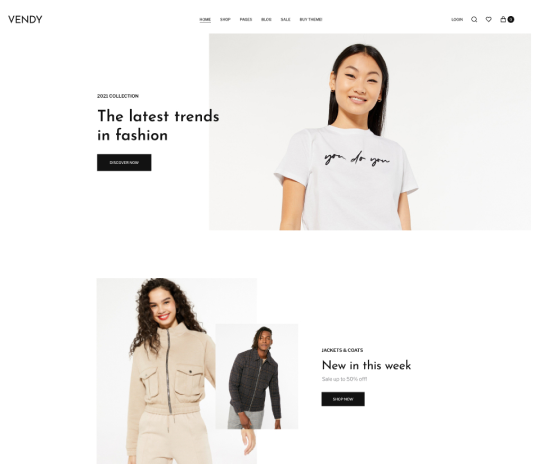The image showcases the homepage of a shopping website named "Vendee," visible in the top bar and navigation bar. Prominently on the top left, the word "Vendee" is displayed. Centered on the page are various navigation tabs, although the text is quite small and hard to read. The tabs include: "Woman," "Shop," "Pages," "Blogs," "Sale," and an enthusiastic "Buy Them!" On the right side of the navigation bar, there is a text that reads "Log In," followed by a search magnifying glass icon, a heart icon, and a shopping bag icon with a black circle containing the number three inside it.

Below the navigation bar, on the right side, an Asian woman is featured wearing a shirt with the cursive text "You do you." Opposite her, the text "2020 Collection" and "The latest trends in fashion" is displayed. Beneath this text, there is a black box with white lettering that says "Discover Now."

Further down the page, another photograph features a smiling Hispanic woman with curly hair, light skin, and bold red lipstick. She is clothed in a canvas shirt and pants. To her right, there is a smaller image of a black man with curly hair, dressed in a black blazer and white shorts, leaning slightly to the side. Accompanying this image is the text "Jackets and Coats, New in This Week," followed by faint gray text stating "Save Up to 50% Off." Below this, there is another black box with white text that says "Shop Now."